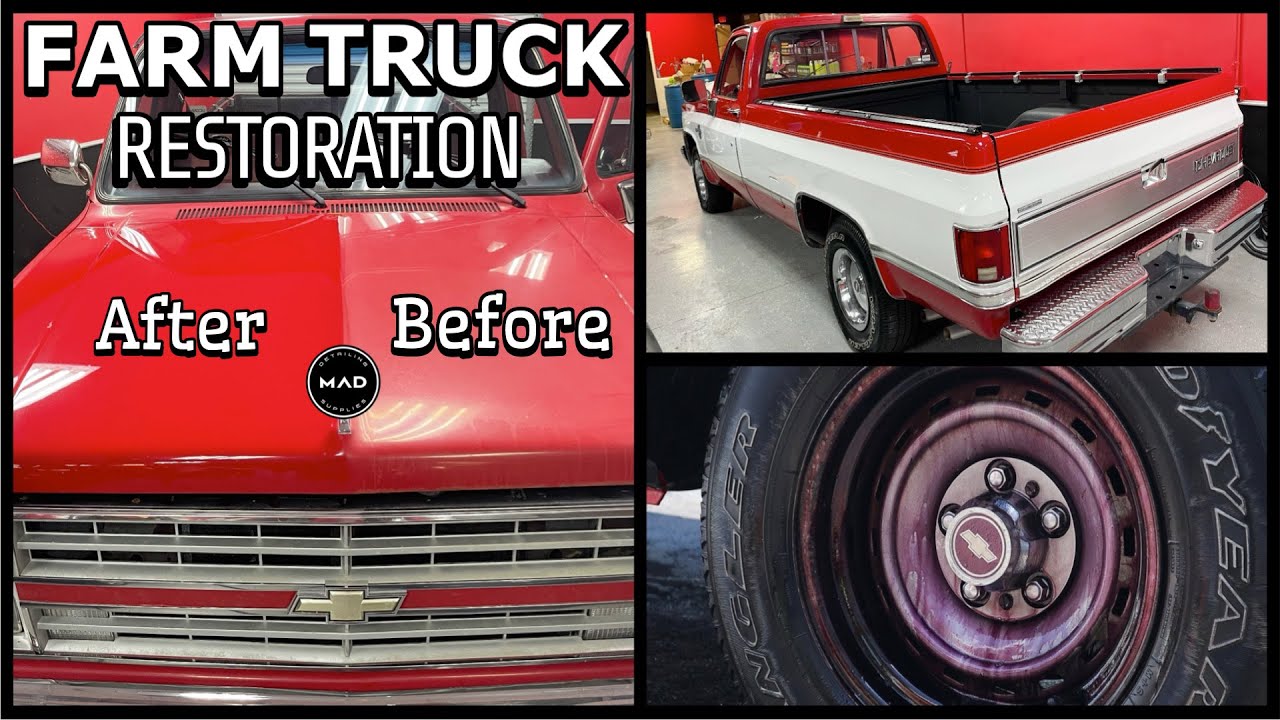The image showcases a detailed "Farm Truck Restoration" with a clear emphasis on the transformation of a Chevrolet truck. The restoration process is depicted with three distinct sections. On the left side, there are before-and-after images of the front of the truck, highlighting a transition from a sun-bleached, faded red to a vibrant and bright red. The truck's front, facing forward, features a silver grille with two red stripes, one aligned with the Chevrolet symbol and another beneath it.

Centered text at the top reads "Farm Truck Restoration" in bold white with a black outline, and just below it, "After" and "Before" are juxtaposed in the middle. Above the truck's hood, a black circular emblem says "MAD" in white text.

In the top right section, another image shows the truck's full body, sporting a red color with distinctive white stripes along its side and back. Below this image, the bottom right displays a close-up of a black Goodyear tire with greasy details, illustrating the thorough and greasy nature of the restoration work.

Collectively, the images and text underscore the meticulous transformation of this classic farm truck from its original worn state to a revitalized, vibrant vehicle.